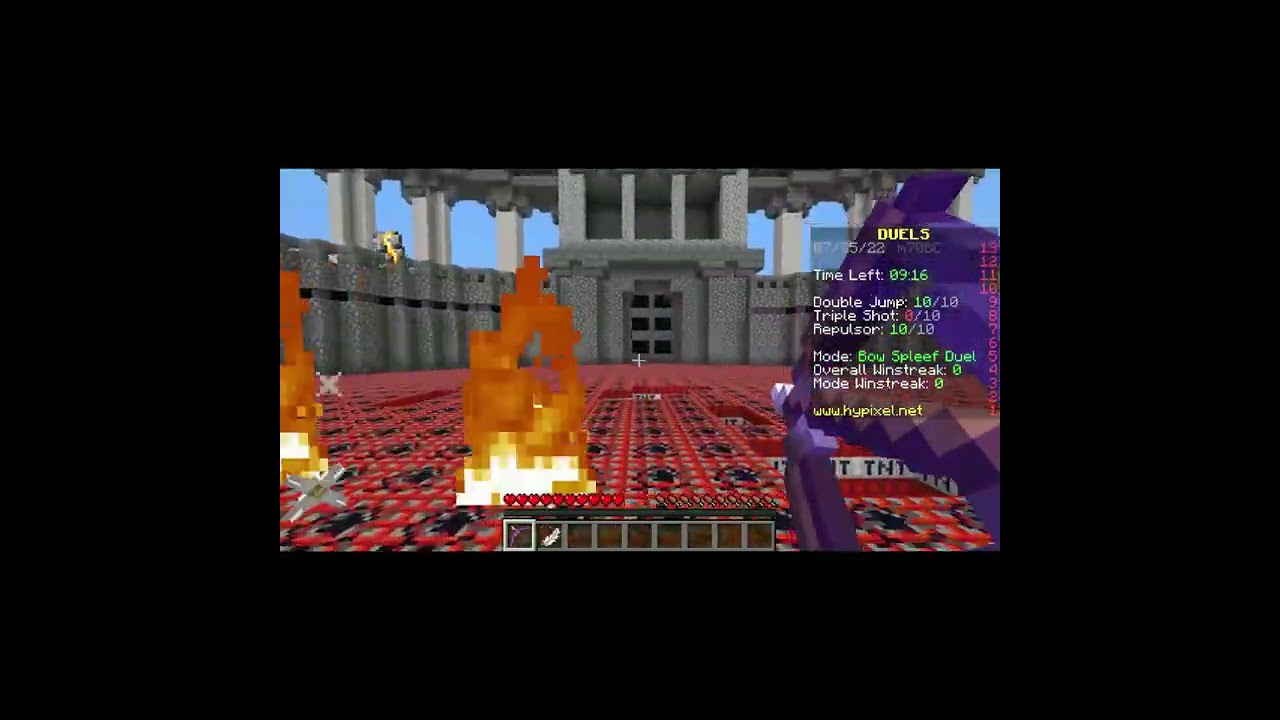This detailed still image, appearing to be a pixelated screenshot from the Minecraft video game, features a vibrant and dynamic scene filled with distinct elements. The primary focus is a floor heavily laden with dynamite, positioned centrally in the image. The background displays a large stone building stretching towards the left, framed by a solid black border. In the foreground, a long carpet composed of red, white, and black runs across the scene, with noticeable sections of red and white flames and indistinguishable purple areas to the right.

The image is punctuated with crucial game interface elements. Central text includes "Duels," a countdown timer showing "9 minutes 16 seconds left," and various game statuses: "double jump (10/10)," "triple shot (0/10)," and "repulsor (10/10)." Other text elements include gameplay modes such as "bowspleef duel," and tracking statistics like "overall win streak" and "mode win streak," both currently at 0. The onscreen URL www.highpixel.net is faintly visible, and a brown icon bar at the bottom features small square cells for tool and option selections.

The color palette of the scene is rich and varied, with shades of black, blue, gray, orange, yellow, purple, and red adding depth and contrast to the dynamic in-game environment.